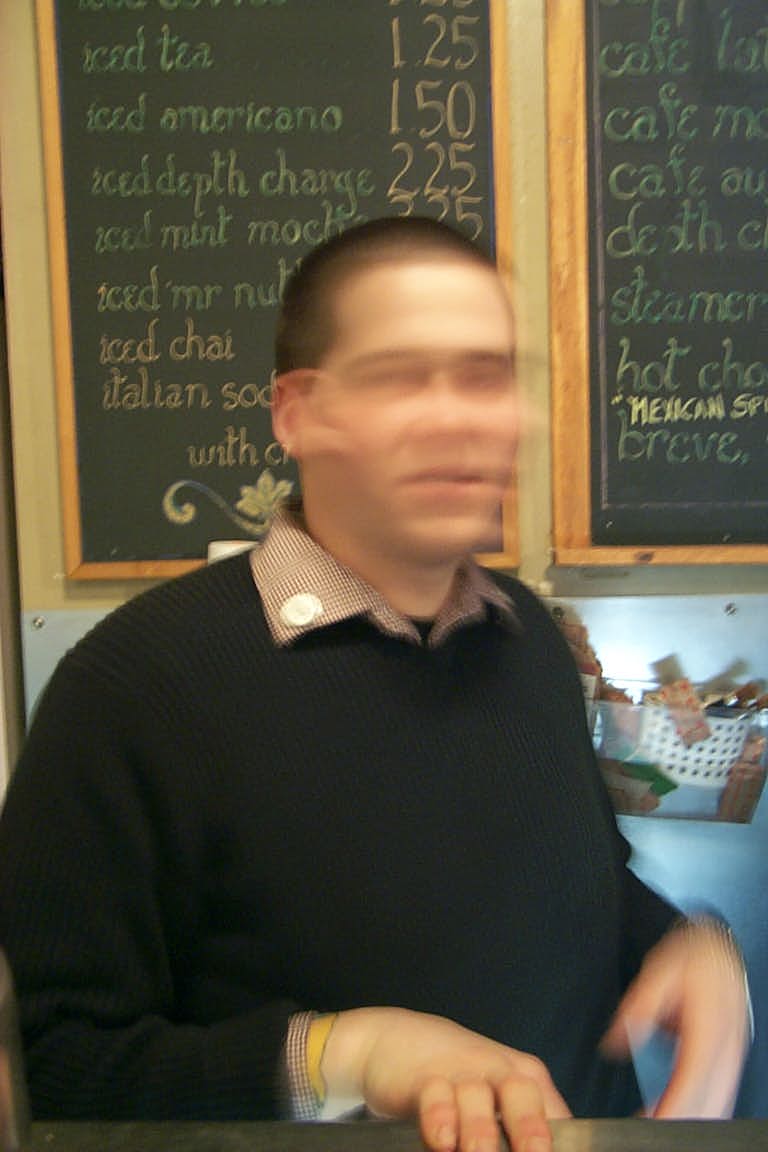In this photograph, a middle-aged man is centrally positioned, facing the camera with a slightly blurred and indistinct facial expression, indicative of movement from right to left. He is dressed in a black, wool-like sweater, beneath which a collared shirt is visible. The collar of the shirt protrudes from the neckline of the sweater. He appears to be seated at a table, with his right hand resting on its surface and his left hand raised and positioned near his stomach. The man has very short black hair. The background reveals a cozy coffee shop setting, with a dark green chalkboard displaying various coffee items and their prices.